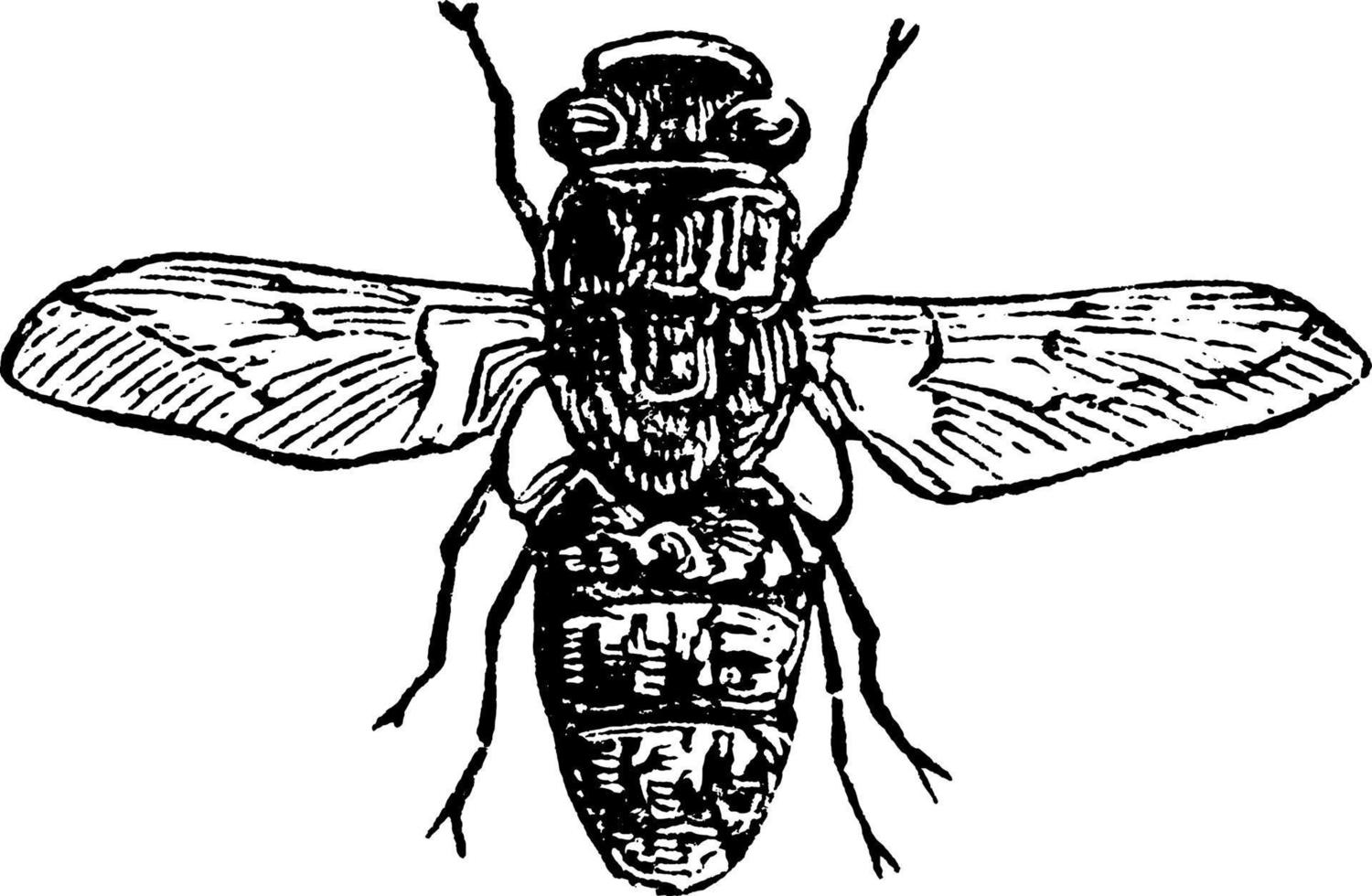This image is a detailed, black and white, hand-drawn depiction of a large insect, likely a fly, presented against a solid white background. The drawing appears to have been printed, giving it a crisp, replicated look. The fly is illustrated from an overhead perspective, showcasing its intricate features. Its head is positioned at the top of the image, featuring prominent, bulging eyes that have a slightly iridescent quality. Two front legs extend upwards on either side of the head, and these legs, along with the two rear legs pointing backward, culminate in forked, two-pronged tips.

The elongated thorax of the fly is segmented into three distinct sections that decrease in size towards the round end of the abdomen. The wings, extending from the sides, are long and narrow, adorned with detailed sketching that includes diagonal lines along the edges and horizontal lines within, suggesting translucence. The overall presentation is clean, with no additional text or borders, allowing the viewer to fully appreciate the meticulous artistry of the insect's form.